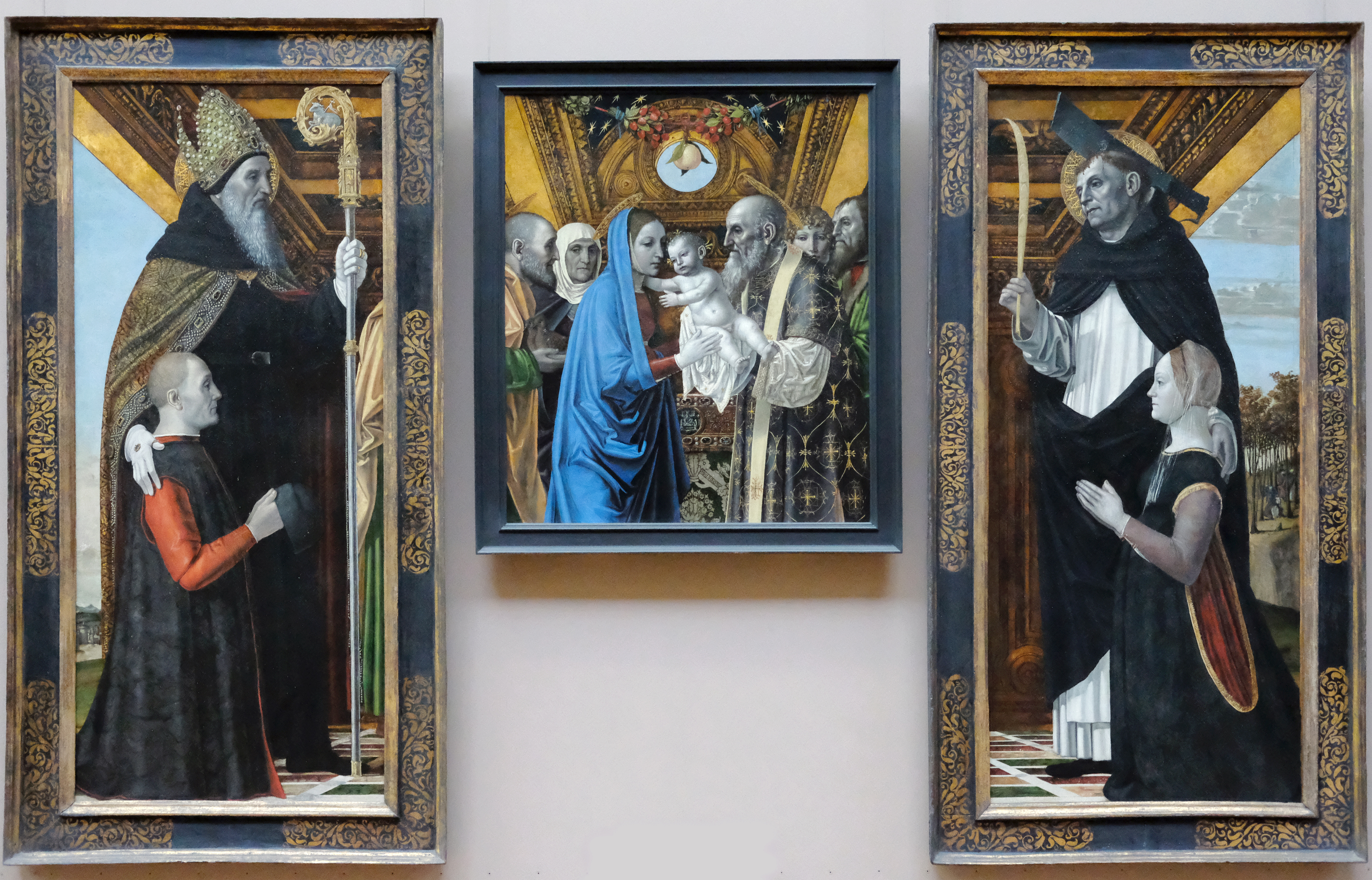The image consists of three distinct, centuries-old religious paintings arranged on a wall. The central painting, which is almost square, depicts Mary in a striking blue robe holding baby Jesus, with an older man, likely Joseph, and other figures present, probably representing a biblical scene surrounded by reverent onlookers. The paintings flanking the centerpiece are rectangular and feature religious ceremonies. 

On the left, a larger man dressed in a gold and black cape with an elaborate gold headpiece, possibly a Pope or high-ranking church official, stands with a staff and places his hand on the shoulder of a kneeling man wearing a sleeveless black gown over a copper-colored shirt, set against a backdrop of gray, blue, and yellow hues. This conveys a scene of solemn prayer or blessing.

The right painting portrays another religious figure, holding a ceremonial wand, placing his hand on the shoulder of a kneeling woman with her hands clasped in prayer. These side paintings emphasize the devotion and piety directed towards the central depiction of Mary and Jesus, encapsulating a rich tableau of historical and religious reverence.